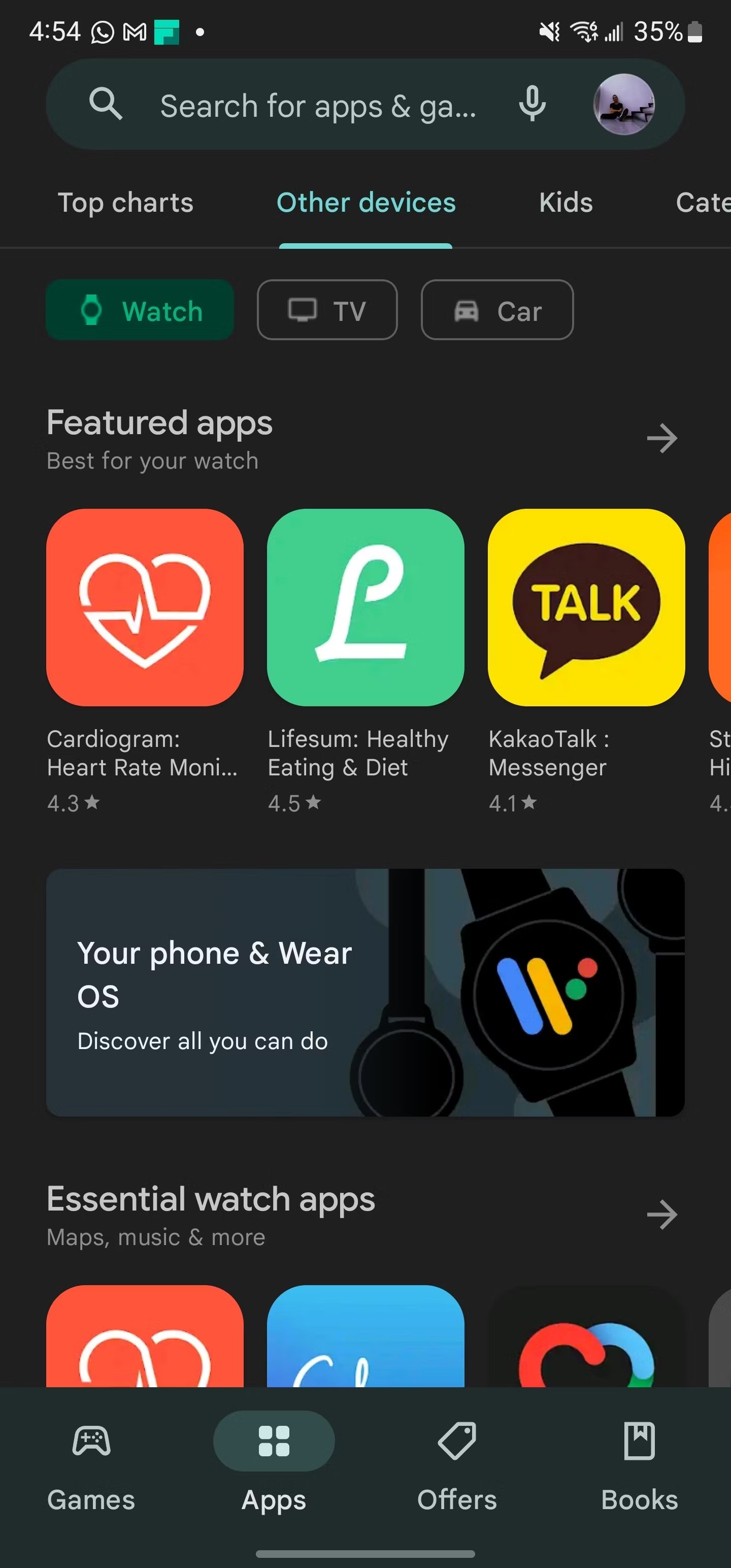This is a detailed caption of the screenshot described:

---

The screenshot captures a section of an app store interface. The screen displays a header indicating "454" and "35%" along with a search bar that partially reads "search for apps and games ga...". Below the search bar are several categories including "Top Charts", "Other Devices", "Kids", with "Other Devices" underlined. 

The interface is segmented into various sections such as "Watch", "TV", "Car", "Featured Apps", and "Best for You". Featured apps shown include "Cardiogram", "Lifesum: Healthy Eating and Diet", and "KakaoTalk Messenger". Beneath the "Your Phone and Wear OS" section is a prompt to "Discover All You Can Do", with a suggestion for "Essential Watch Apps", accompanied by an arrow pointing to the right.

Toward the bottom, the categories "Maps", "Music", and "More" are listed. Finally, at the very bottom of the screen, tabs display options including "Games", "Apps" (highlighted with a gray rectangle as the selected tab), "Offers", and "Books." The bottom middle area of the screen has a light gray background.